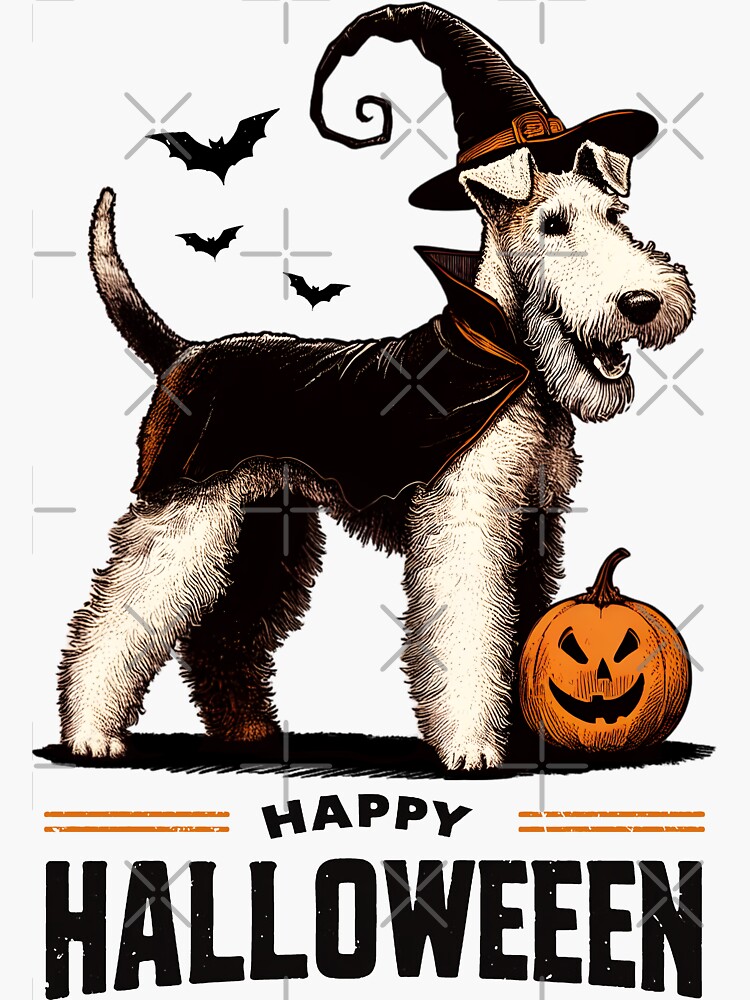This detailed illustration features a Jack Russell Terrier-like dog with a long face and slightly bent ears, predominantly white with light cream fur accented by brown patches on its nose and under its ears. The dog is dressed as a witch, wearing a black witch hat with an orange belt buckle, its tip spiraling whimsically. Complementing the hat, the dog dons a black witch cape with a high, orange collar. The canine appears to be posing, with a black shadow in the foreground adding to the visual depth. Surrounding the dog are three flying black bats placed toward the top left of the image. A jack-o-lantern with a carved face sits at the bottom right. The background is white with decorative X's and plus signs resembling watermarks scattered throughout. Below the dog, in an arched and somewhat vintage-styled font, "Happy Halloween" is inscribed in capital black letters. The overall design suggests a festive, Halloween-themed cartoon or inked art piece.